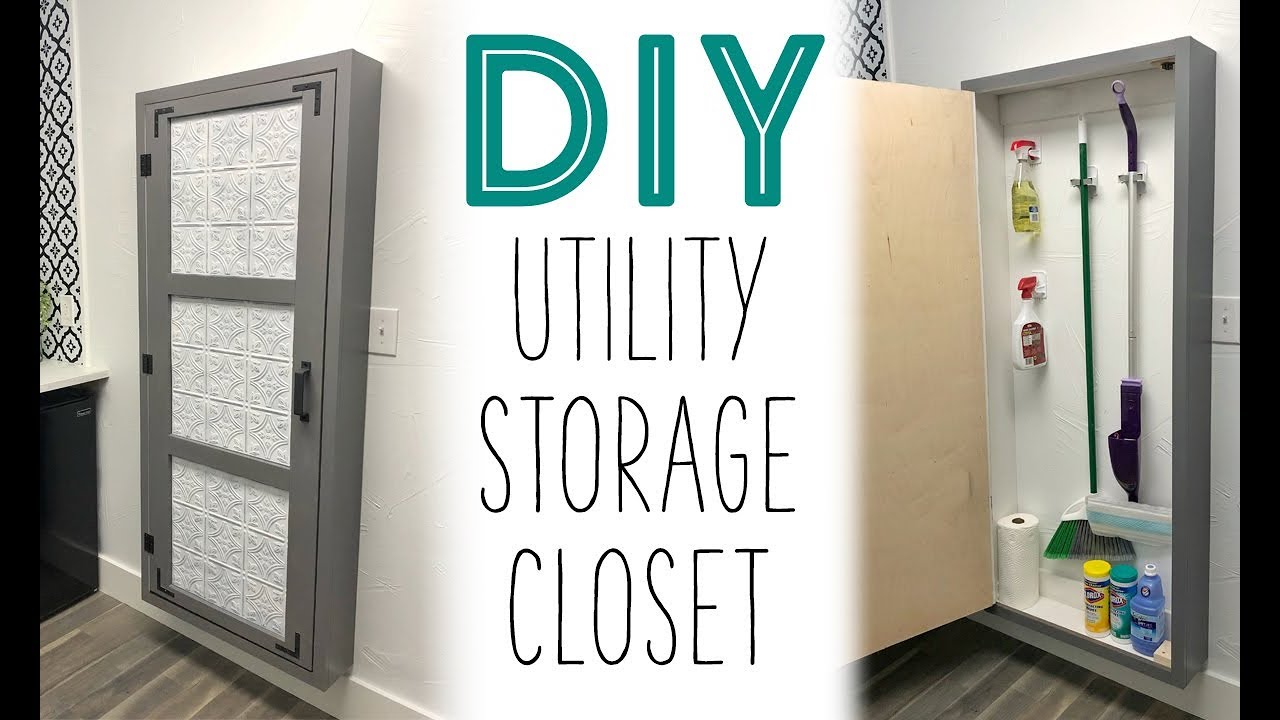The image showcases a DIY utility storage closet with a central text area displaying "DIY Utility Storage Closet." The DIY text is prominently featured in green with a white 'D' inside a larger green 'D,' while the words "Utility Storage Closet" are written in thin black lines. On the left side of the image, the closed gray utility closet features three square panels, black handles, and black hinges, and is placed beside a kitchen cabinet. The floor beneath the closet is gray and wooden, and the white walls surrounding it have a decorative black circular and triangular pattern. On the right side, the same closet is shown open, revealing various cleaning supplies neatly organized inside, including Clorox wipes, a Swiffer, Swiffer solution, paper towels, a broom, sprays, and a mop. The detailed juxtaposition effectively highlights the practical storage capabilities of the DIY utility storage closet.